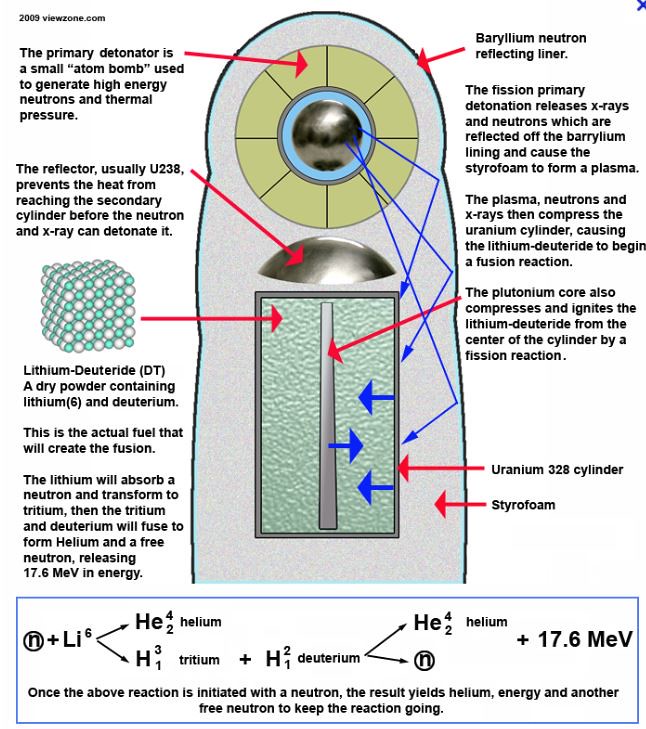The image is an educational poster illustrating the intricate components and reactions involved in the detonation of a nuclear bomb. Dominating the center of the diagram is the primary detonator, a small atom bomb designed to generate high-energy neutrons and thermal pressure. Surrounding this central bomb are several labeled parts with red arrows pointing to each, indicating the step-by-step process of the detonation sequence.

At the core of the diagram, a metallic orb represents the plutonium core, which compresses to ignite the lithium deuteride in the center of the cylinder during the fission reaction. A beryllium neutron reflecting liner surrounds the core, aiding in reflecting X-rays and neutrons which are crucial for initiating the subsequent fusion reaction.

The poster highlights the use of a U-238 reflector to prevent heat from reaching the secondary cylinder before the neutron and X-ray can initiate detonation. The essential compound, lithium deuteride (DT), a dry powder, is noted as a critical fuel that absorbs neutrons to transform into tritium. The fusion of tritium and deuterium results in the release of helium, energy, and another free neutron, perpetuating the reaction cycle.

Additional details include a series of equations at the bottom of the poster, elucidating the scientific basis of the reactions. The visual aid is decorated in a palette of black, white, dark blue, light blue, gray, olive, silver, and green and yellow accents, providing a clear and visually engaging explanation of the nuclear detonation process. The top left corner of the image features the source text, "2009viewzone.com."

Overall, this poster serves as a comprehensive educational tool detailing the complex chemical and physical reactions governing the detonation of a nuclear bomb through precise diagrams, highlighted components, and sequential explanations.